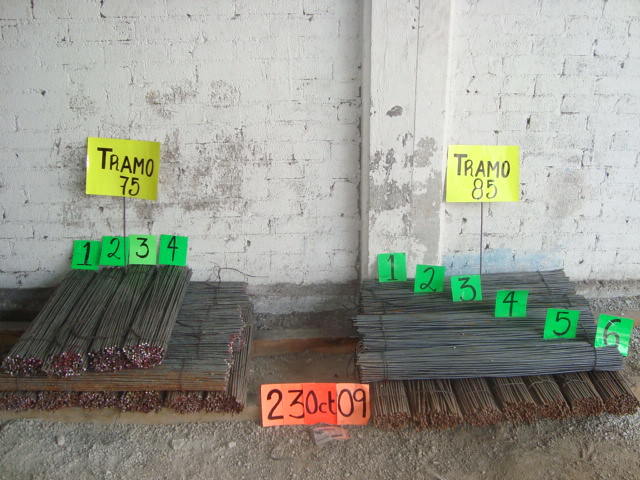The image showcases neatly stacked bundles of rods, possibly rebar used for strengthening concrete, set against a white, faded brick wall in a dusty, gravel-covered area. The top three-fourths of the image prominently feature the back wall, while the bottom quarter displays the gravel floor. The bundles of rods appear in crisscross formations with distinct labels: on the left, a sign reading "Tramo 75" with bundles labeled 1, 2, 3, and another sign above bundles labeled 1, 2, 3, 4, 5, 6 indicating "Tramo 85". These labels suggest sections, potentially in Portuguese. The rods themselves vary in gray and brown hues, complimented by yellow, green, and orange signs with black text. An orange sign with the date "23 October 09" lies at the center on the gravel, further detailing the scene. 

Each side's rows are organized: the right stack comprises one row of rods pointing towards the viewer and another perpendicular one on top. The overall desolate atmosphere, combined with peeling paint on the wall, enhances the industrial and somewhat rustic setting.